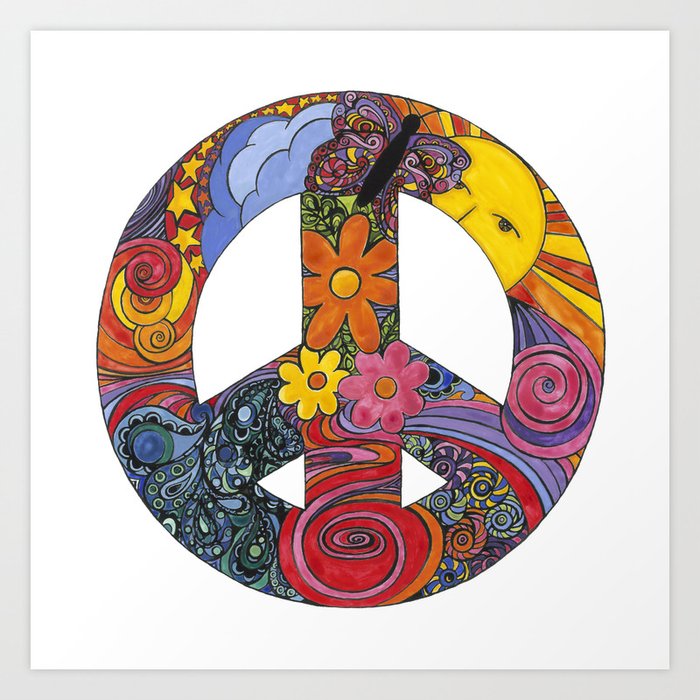This vibrant art piece showcases a multicolored peace symbol filled with intricate and psychedelic designs, evocative of the 60s. Framed in white, the symbol incorporates a wide range of colors including purple, orange, blue, red, pink, yellow, green, and black. Starting from the top, there's a black-bodied butterfly with black antennae and wings adorned with curls in shades of purple, light purple, red, and yellow. Half-hidden behind the butterfly's wing is a serene, yellow sun with a partially visible right eye and extending bursts of red, orange, and yellow rays.

Proceeding clockwise, the artwork features swirling patterns and lines resembling rainbow colors: pink, light pink, purple, light blue, and red. Beneath these are curls of varying colors flowing downward and three flowers arranged vertically—a prominent orange flower with a yellow center, a yellow flower with an orange center, and a pink flower with an orange center. More rainbow lines curve downward at the bottom of the circle, leading towards paisley designs in purple, black, and green. 

Towards the eleven o'clock position, a row of yellow stars set against a red background is followed by a smaller row of red stars on a darker backdrop. This section blends into a series of three fluffy blue clouds, ranging from light blue to darker shades, expanding towards the top. Additionally, two distinctive arrow-like triangles point in opposite directions, contributing to the complex design.

This detailed and colorful composition captures the essence of peace and harmony, blending symbols of nature with vivid, flowing patterns.